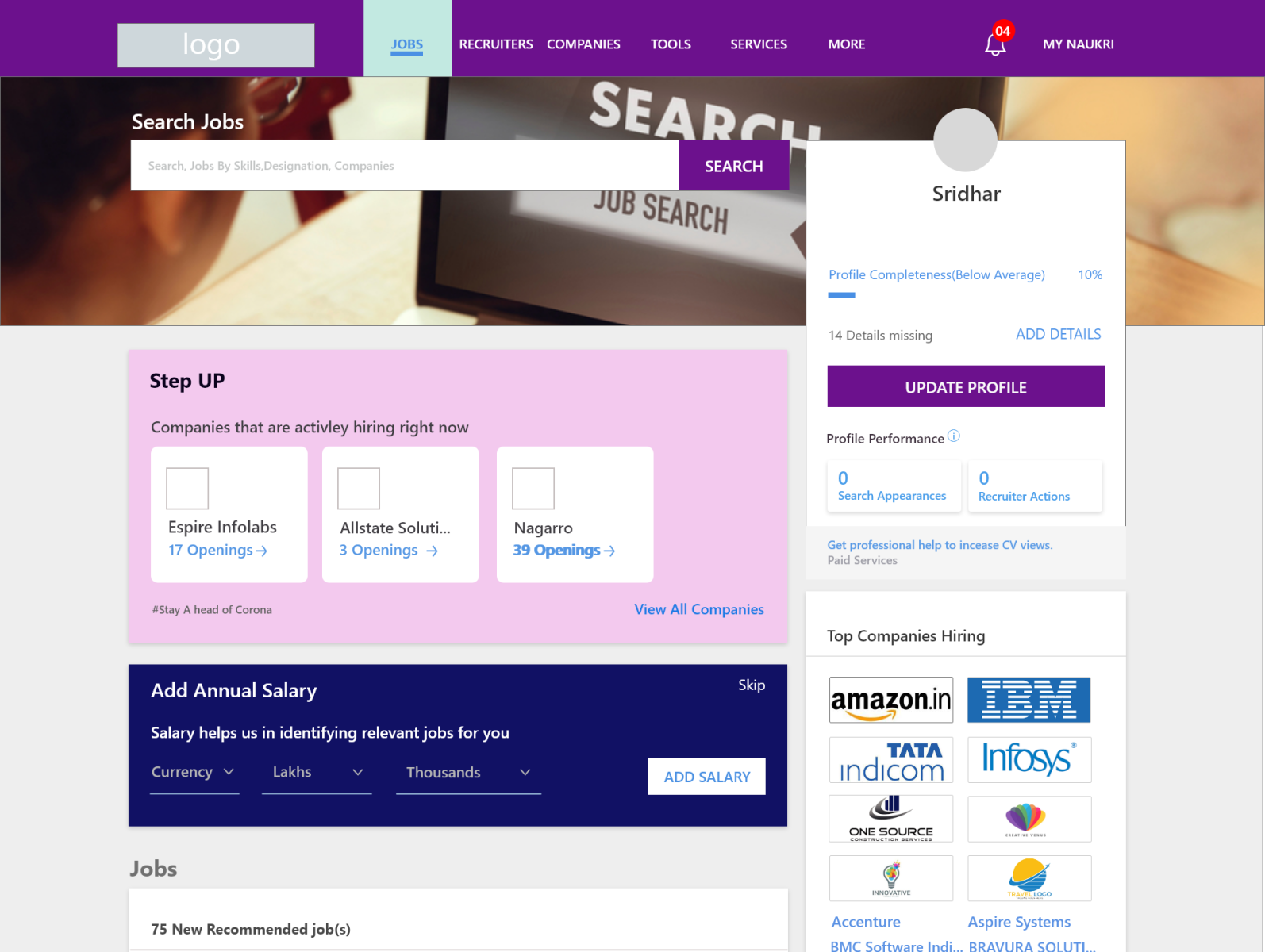A square-shaped screenshot captures a job search website interface. In the upper left corner, there is a rectangular logo icon on a light gray background, with 'Logo' written in white text. To the immediate right, several clickable categories are displayed in white text: Jobs, Recruiters, Companies, Tools, Services, and more. The 'Jobs' category is selected, highlighted with a light blue background, dark blue text, and underlining.

In the upper right corner, the user's name is displayed alongside a bell-shaped notification icon. A small red circular icon with '04' in white indicates four new notifications. The main body of the website consists of large color blocks. Immediately beneath the header with the clickable links, an image depicts a person sitting in front of a computer, actively searching for jobs.

Above the image, a search bar with a white background and gray text reads "Search Jobs by Skills, Designation, Companies." Below it, a pink rectangular button with black text urges users to "Step Up." Furthermore, three square-shaped sections provide additional information about various companies and job openings, with company names and job details written in blue text.